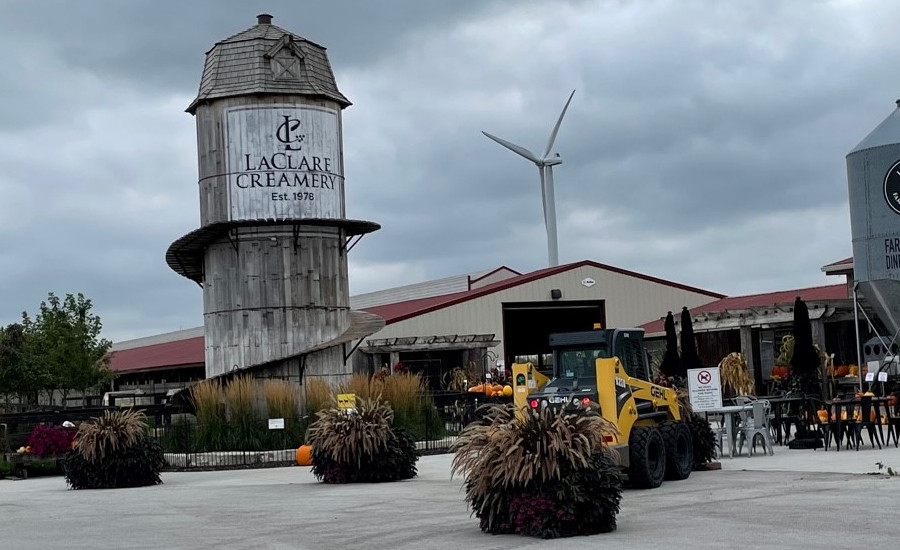This detailed, horizontal outdoor photograph captures the scene outside of La Claire Creamery on a cloudy, stormy day. Dominating the center of the image is a tall, old-fashioned wooden grain tower with a triangular arch-shaped window featuring an X-shaped shutter near the top. Midway down the tower, stairs wrap around it, and a white-painted area reads "La Claire Creamery, established 1978." Scattered in the foreground are three odd black, purple, and beige plants, along with a yellow and black construction tractor. To the right, there are silver and black tables and chairs beneath table umbrellas. A sign that seems to read "no dogs" is partially visible in the background. The setting is framed by large bushes and trees on the sides. Behind the tables, the expansive, one-story creamery building has beige siding and a deep maroon-red roof. The building features multiple towers, including the prominently labeled grain tower on the left and a slightly shorter tower on the right with cut-off text. In the far background, a white wind turbine stands centrally, adding to the industrial feel of the scene.